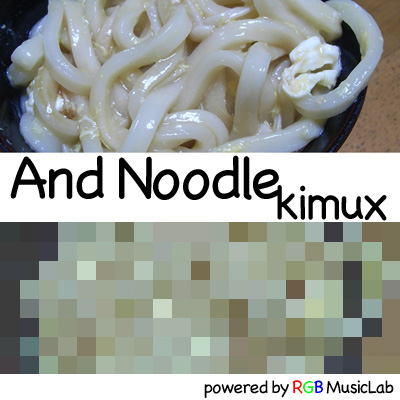The image is a square format, showcasing two distinct sections. The top half features a detailed photograph of white noodles nestled in a black bowl, glistening with sauce or broth, spanning almost the entire frame. The container appears dark, possibly dark blue or black, though the exact color is hard to discern. The background surroundings on the right are medium to dark brown, and on the left, they are dark black, visible only along the edges. In the middle of the image, a white band breaks the visual flow, displaying the text "and noodle KMUX" in bold black letters. The lower half of the image morphs into a highly pixelated version of the noodle photograph above, with blocks of whites, browns, grays, and greens dominating the space. At the bottom right corner of this lower section, the caption "powered by RGB music lab" appears in black text.